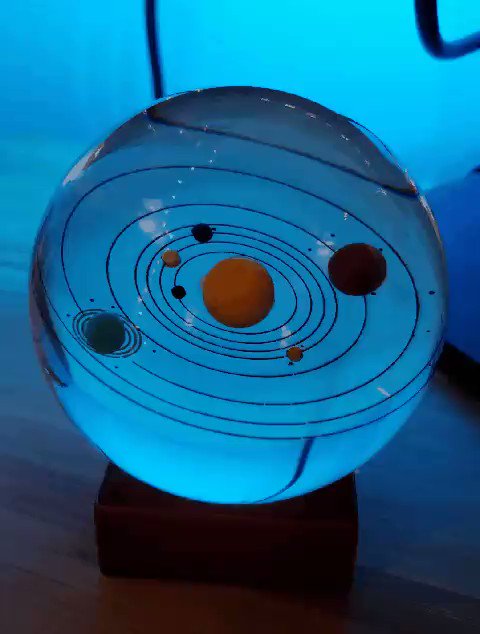The image features a clear glass crystal ball, reminiscent of a fortune teller's sphere, centrally positioned on a natural brown wooden base. The setting appears to be a wooden surface, possibly a desk or flooring, bathed in blue light which creates a soft glow around the ball. Inside the crystal ball is an intricate, miniature replica of our solar system. At the center is the bright yellow Sun, surrounded by concentric rings symbolizing the orbits of the planets. Starting from the Sun, one can see Mercury, Venus, Earth, the red-tinted Mars, followed by a noticeable gap representing the asteroid belt. Beyond the gap, Jupiter is visible, and then Saturn with its distinctive rings and accompanying moons. The sphere displays additional orbital rings, but the planets beyond Saturn are not visible from this perspective. The image is devoid of any text and the dominant colors are various shades of blue, black, gray, orange, red, and brown, all contributing to a visually striking and detailed representation of the solar system. The overall aesthetic suggests it is placed in a bedroom, adding to its decorative appeal.